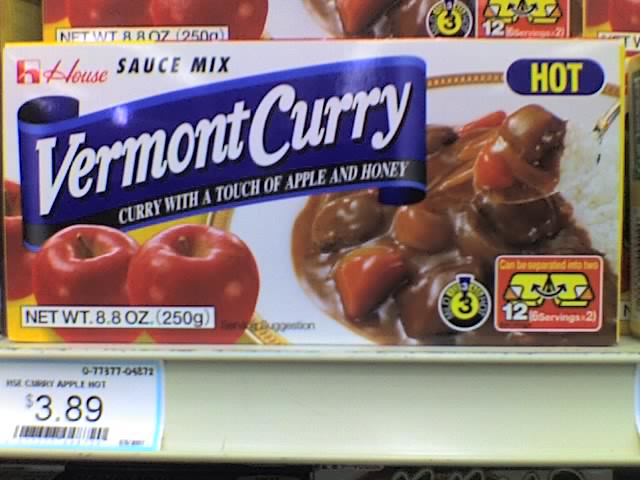This close-up photograph captures a package of Vermont Curry on a store shelf. The package prominently displays the "Vermont Curry" brand logo, with the phrase "Curry with a touch of Apple and Honey" written just below. In the bottom left corner of the package, there are images of two red apples, emphasizing the product's unique ingredients. The main visual in the center-right of the package showcases a plate of rice accompanied by curry sauce and pieces of meat. Near the top left, there is a blue oval with the text "Hot" in yellow lettering, indicating the spice level.

The bottom right corner features a red box suggesting that the package contains "two yellow packages" inside. The net weight of the product, 8.8 ounces (250 grams), is also clearly marked on the package. Below the package on the white shelf, there is a price tag displaying $3.89 along with a barcode. In the background, you can partially see another curry box above this one, indicating that the shelves are well-stocked.